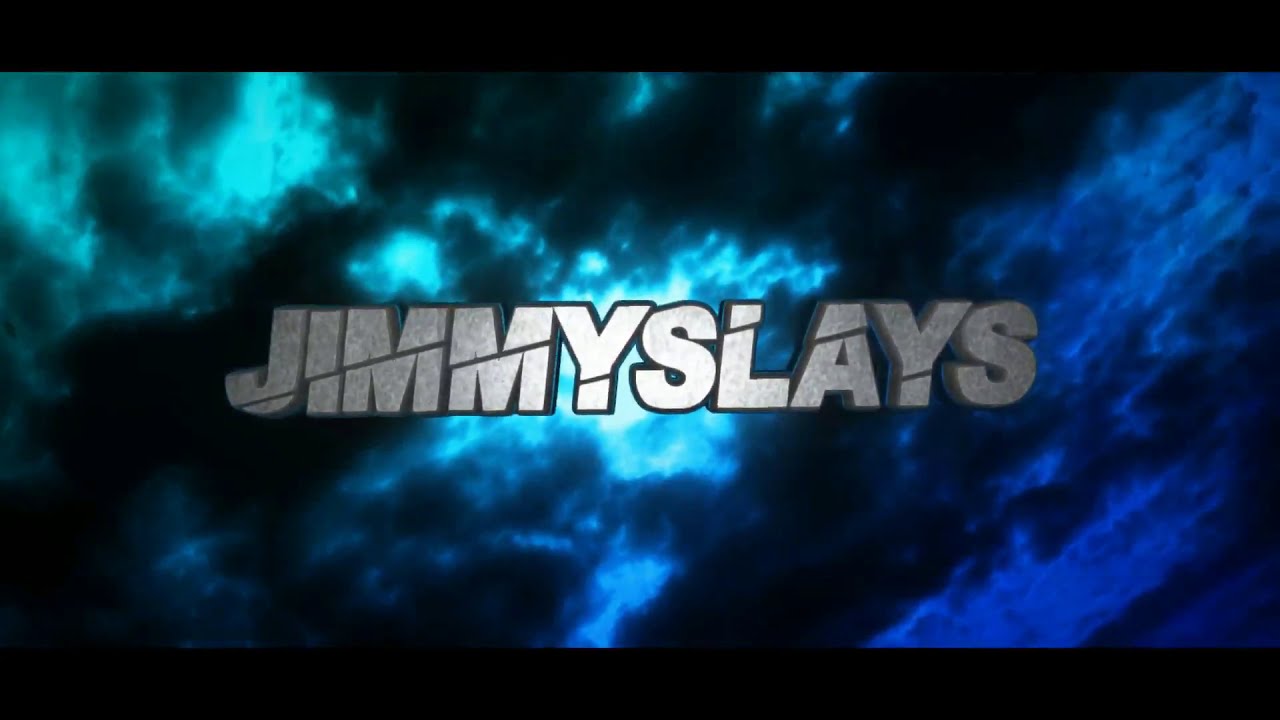The image appears to be a title screen for a video, possibly for a streamer named Jimmy Slays. The background is a dramatic, stormy sky featuring dark clouds illuminated by brilliant, electric blue light, giving the impression of lightning piercing through storm clouds. Predominantly, the color scheme is black and various shades of blue, transitioning from turquoise on the left to a vibrant violet-blue on the right. Thin black rectangles frame the image on the top and bottom edges.

Foremost in the image is the name "JIMMY SLAYS," written in a bold, three-dimensional metallic font. The letters have a gradient effect, with the center of the text illuminated as if by a white light, fading into darker shades of gray toward the edges. Each letter appears to be crafted from pieces of metal with oblique, sword-like slices adding dynamic detail across them, resembling a samurai sword chop. This slicing effect is particularly prominent on letters J, I, M, M, Y, L, A, and Y. The text is further defined by a black outline, enhancing its visibility and giving it an aggressive, high-energy appearance fitting for a gaming or streaming brand.